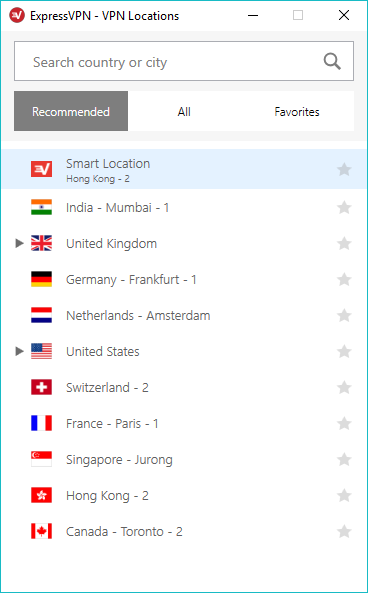This image depicts the server location selection menu within the ExpressVPN application. At the top of the menu, there's a search box labeled "Search country or city" which allows users to quickly find specific VPN locations. The menu is currently set to display "Recommended" locations, highlighting the most optimal servers for the user. Additional categories available include "All" and "Favorites," the latter of which stores previously marked VPN locations.

In the recommended list, notable server locations include Smart Location in Hong Kong, Mumbai in India, and various cities in the United Kingdom, which can be expanded into more options via a drop-down menu. Similarly, the United States has a drop-down menu revealing multiple server choices. Other recommended locations feature Frankfurt in Germany, Amsterdam in the Netherlands, Toronto in Canada, Paris in France, Jurong in Singapore, as well as additional servers in Hong Kong.

Each country in the list is accompanied by its national flag, providing visual cues for easier identification. To the right of each location, there is a star icon that users can click to add that server to their "Favorites," facilitating quick access in the future.